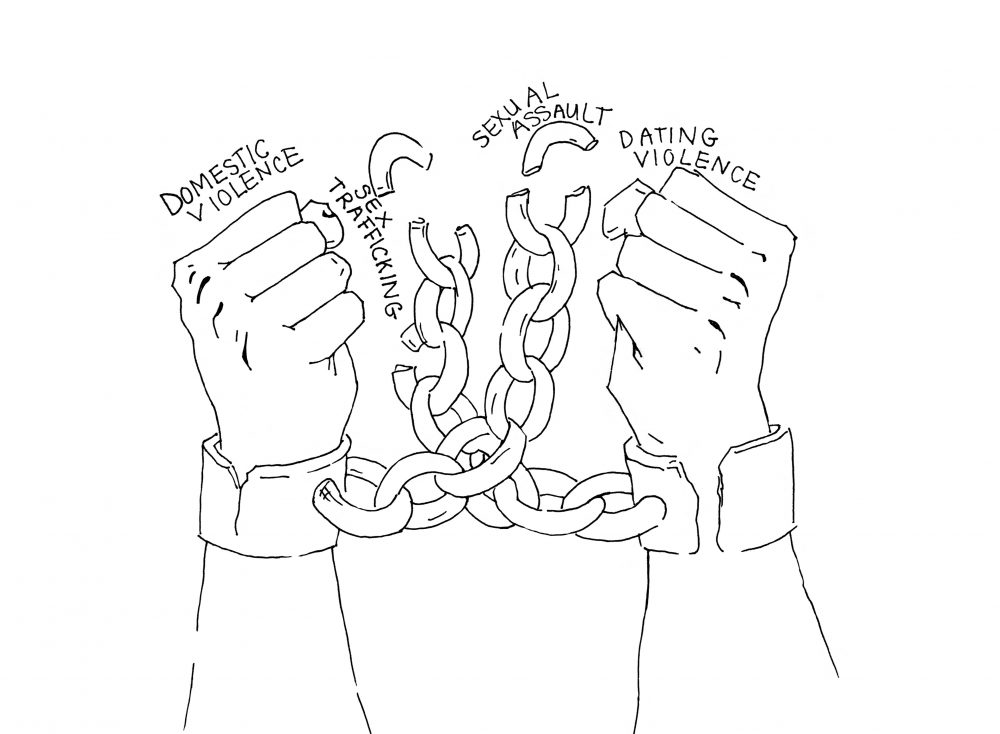This black-and-white illustration prominently features two forearms ending in clenched fists, which are bound by shackles and chains. The illustration is simple, focusing on the essential elements with minimal detail. The chains connecting the shackles are broken, signifying a sense of breaking free. The left shackle is completely cracked, while the right shackle is shown with a significant crack, further emphasizing the theme of liberation. Surrounding the fists are words related to various forms of abuse: "Domestic Violence" curves around the left fist, "Sex Trafficking" is placed near the middle, "Sexual Assault" arcs around one of the broken chain links, and "Dating Violence" sits above the right fist. These words are all rendered in black. The lack of intricate details like fingernails contrasts with the clear depiction of the knuckles and the forceful image of the broken chains and shackles.